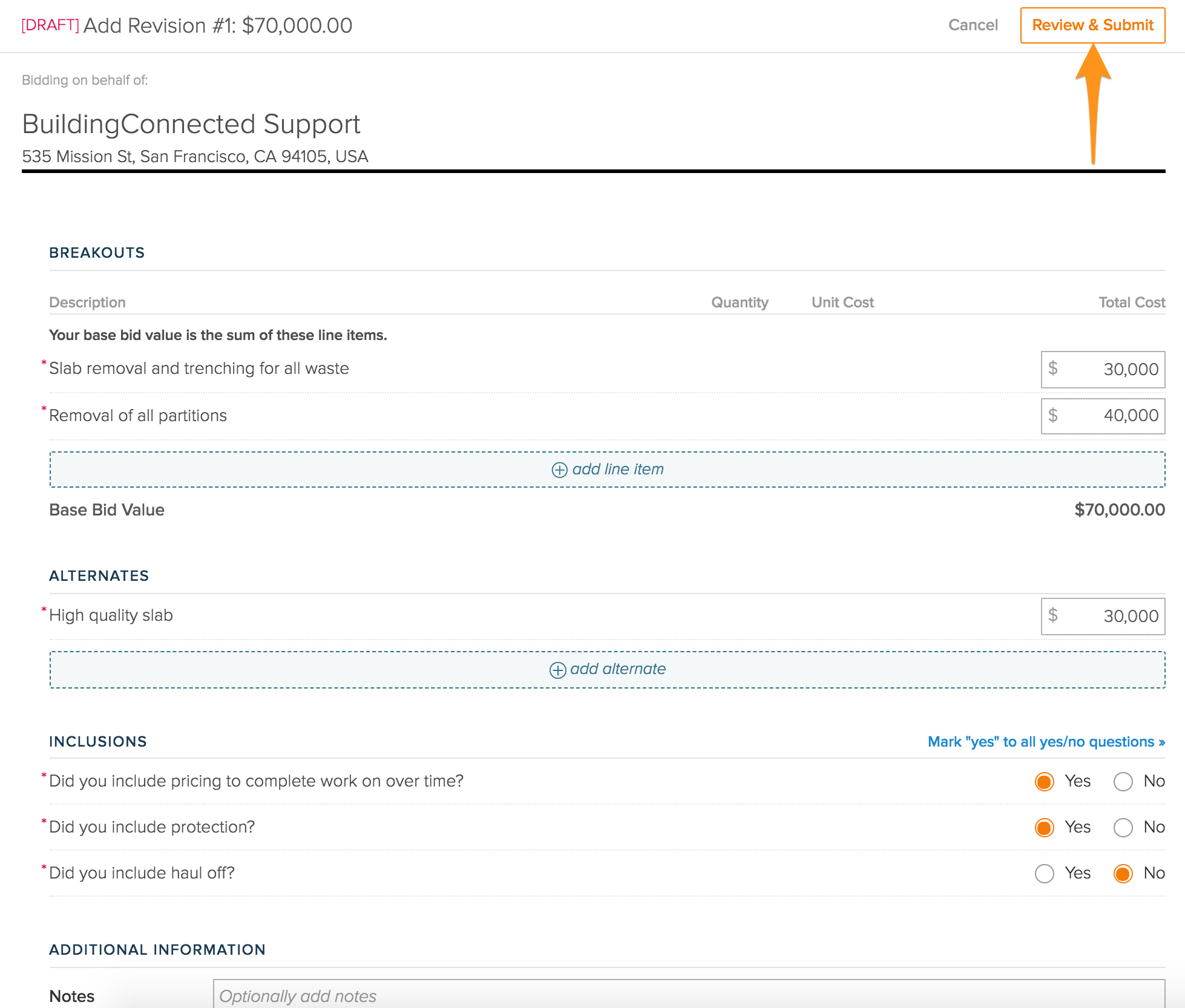This screenshot depicts a detailed draft budget displayed on a computer screen, set against a white background with predominantly black text. At the top, the word "Draft" is highlighted in a pinkish-red color, signifying its status. Following that, it mentions "Add Revision Number: 170,000." On the top-right corner, there are options for "Cancel," "Review," and "Submit," the latter two encapsulated within an orange rectangle and accompanied by an upward-pointing orange arrow.

Below this section, the screen features "Building Connected Support," including an address located in San Francisco, California. A horizontal black line spans the width of the page beneath this section. The next line introduces the category "Breakouts," with subsequent subcategories listed under it. On the right side, the "Breakouts" section details two cost entries: one totaling $30,000 and another $40,000.

Further down, a prominent blue rectangular button offers the functionality to add additional information. Following this, an "Alternatives" section is presented, which includes another cost entry of $30,000 and the option to add more items. The subsequent "Inclusions" category features a series of yes-or-no options, with selected choices encircled in orange.